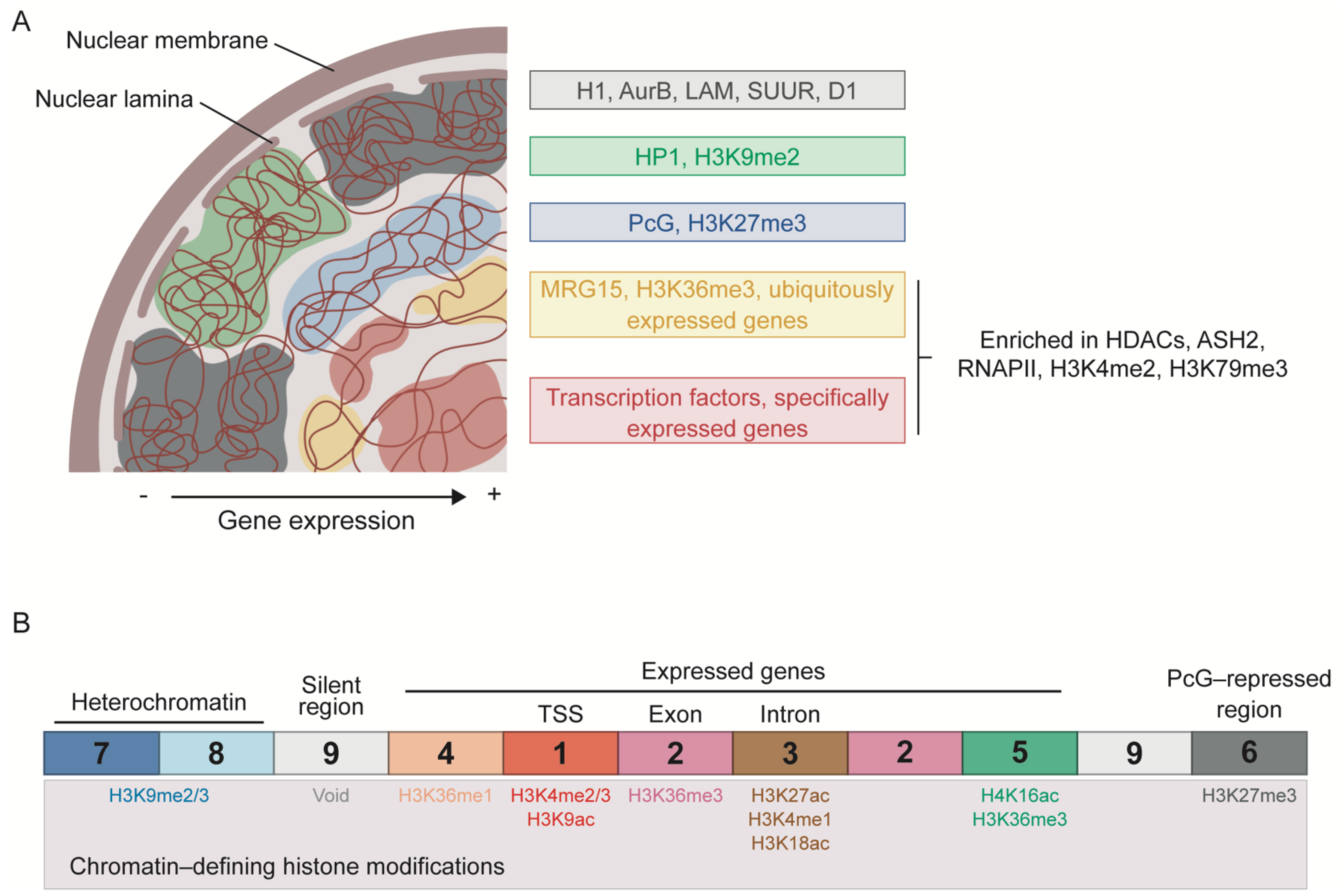The photograph depicts a highly detailed chart from a science textbook, illustrating cellular structures and gene expression mechanisms. In the upper left corner, labeled "A," there is a semi-circular image representing part of a cell. The outer gray edge is identified as the nuclear membrane. Inside this semicircle, a variety of colored blobs—green, blue, yellow, and peach—are scattered, overlain with brown and red squiggly lines labeled as the nuclear lamina. Underneath this section, the text reads "gene expression," indicating the functional focus of this part of the diagram.

To the right of this image are multiple colored rectangles in a sequence of black, green, blue, yellow, and red, each containing scientific labels with combinations of letters and numbers. A particular set of rectangle labels includes "transcription factors" and "specifically expressed genes," emphasizing important cellular components. Additional annotations to the right mention "enriched in HDACs" alongside more alphanumeric codes.

At the bottom of the chart, labeled "B," is another segmented section that provides data on chromatin structure and histone modifications. This part features numbers arranged as 7, 8, 9, 4, 1, 2, 3, 2, 5, 9, 6, each number set against colorful backgrounds—in shades such as different blues for 7 and 8, white for the 9s, and pink for the 2s. These segments are subdivided into color-coded regions with labels like "heterochromatin," "silent region," and "PCG repressed region." At the bottom left corner of this section, the caption reads "chromatin defining histone modifications," providing a clear summary of the depicted modifications and their chromosomal locations.